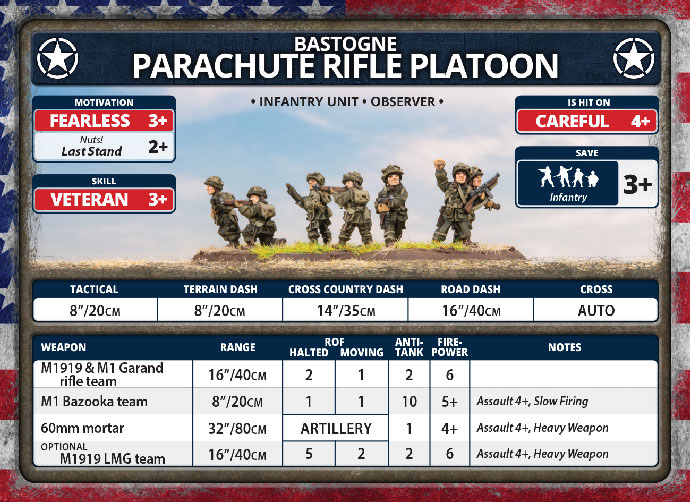The image is a highly stylized graphic featuring a parachute rifle platoon infantry unit, set against a distressed American flag background with patriotic colors and star elements. Dominating the top is the text "BASTOGNE Parachute Rifle Platoon" in large capital letters on a dark blue rectangle. Below this are cartoon-style illustrations of seven soldiers, some facing forward and others turned away, stationed against a blue sky and standing on a grassy ledge.

Surrounding the soldiers are various stat boxes and descriptive text. On the left, the image details the unit's capabilities with phrases like "Motivation: Fearless 3+", "Nuts: Last Stand 2+", and "Skill: Veteran 3+" in multicolored red, white, and blue boxes. On the right, additional stats read "Is Hit On: Careful 4+" and "Save: Infantry 3+". A large white rectangle at the bottom provides similar information, along with mention of various weapons, ranges, and ratings, and notes about slow firing or heavy weaponry.

The true nature of the image is ambiguous, leaving it unclear whether it refers to a real military unit or a virtual entity from a game or competition. The central visual is anchored by the soldiers, but the text also references a cross-country dash and different terrains, further contributing to the uncertainty about its authenticity.